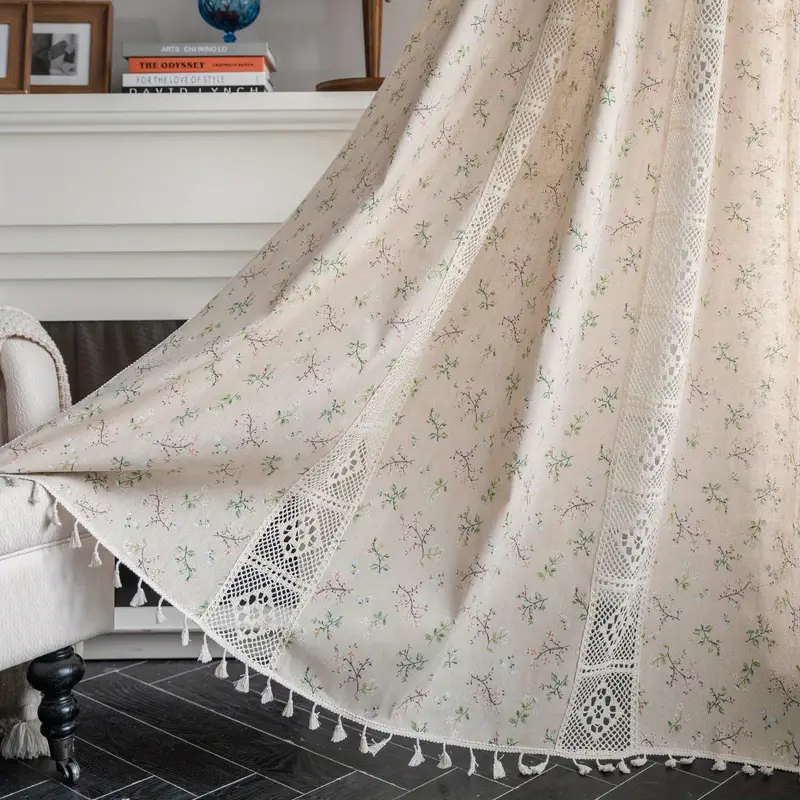The image captures an elegantly decorated home interior, featuring a large, white drapery that cascades from the upper right corner and extends outwards to the left center. The bottom of the drapery is adorned with intricate tasseled fringes and lace accents, showcasing delicate floral patterns and stems in shades of light green, blue, and black. A portion of the drapery drapes over a cushioned chair with black legs, prominently positioned on the right side of the image.

In the background, on the left, stands a molded mantle of a fireplace topped with a candlestick. The mantle is detailed with molding at both the top and bottom, enhancing its classic look. To the right of the mantle, a white shelf holds a collection of books, wooden-framed pictures, and a small globe. The floor beneath is made up of shiny, black rectangular marble tiles. The scene is well-illuminated, highlighting the details and creating a bright and clear setting.